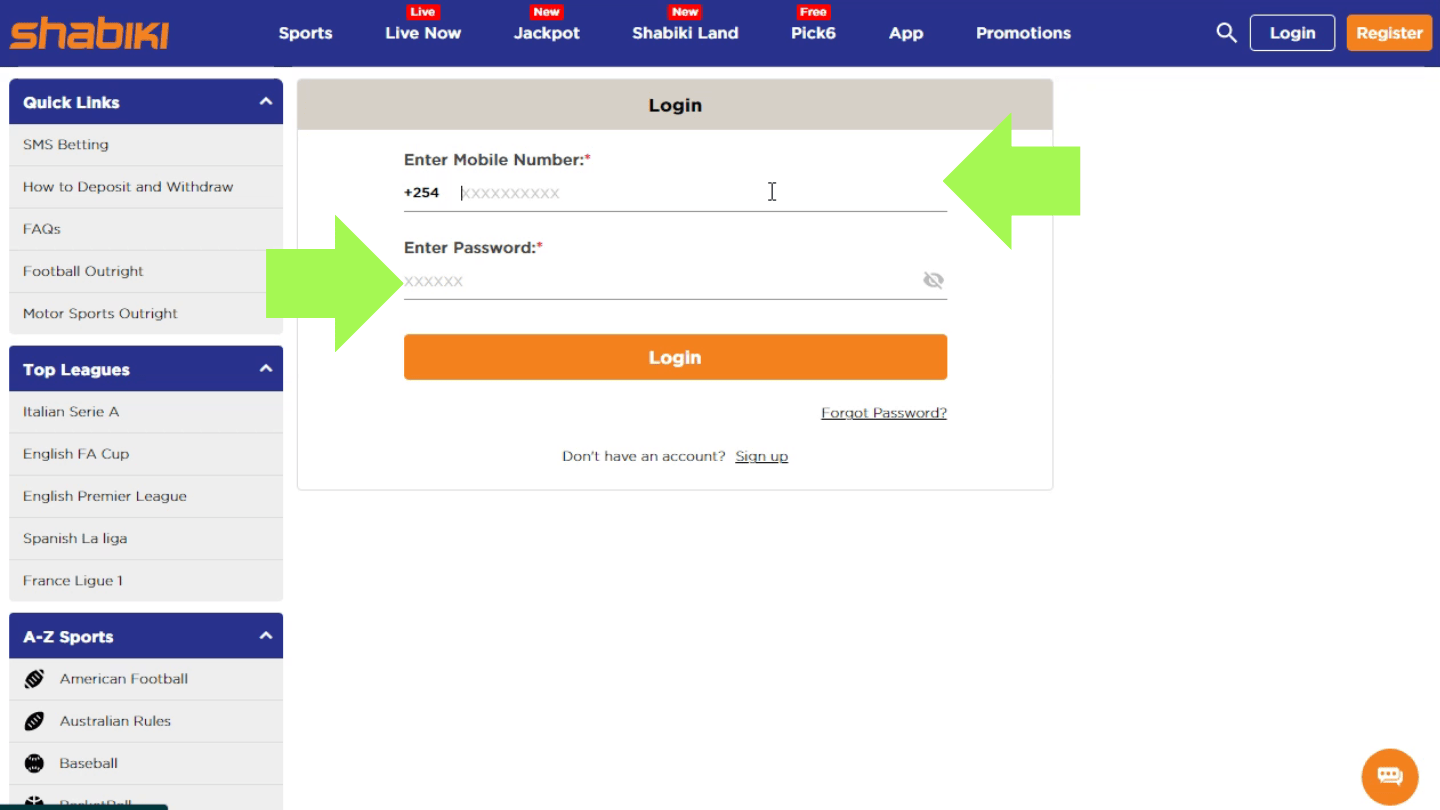A screenshot of a website featuring a straightforward design. The page is topped with a blue banner, bearing the site name "Shabiki" in vibrant orange font on the upper left. Adjacent to this name, navigation categories are listed in white font, including Sports, Live Now, Jackpot, Shabikiland, PickSix, App, and Promotions. Towards the right side of this banner, there is a search bar followed by a blue login button and an orange register button.

Below the blue banner, in the main white section of the page, there is a login screen prompting users to "Enter Mobile Number" with a prefilled country code (+254) and an "Enter Password" field, each marked by green arrows pointing towards them. An orange login button with white text is positioned below these fields.

On the left-hand side of the page, a vertical navigation menu lists quick links and categories for users to explore. These include Quick Links, SMS Betting, How to Deposit and Withdraw, FAQs, and sections like Football Outright, Motorsports Outright, Top Leagues, Italian Series A, English FA Cup, English Premier Cup, Spanish La Liga, France League One. Further down, an A to Z Sports list features American Football, Australian Rules, and Baseball.